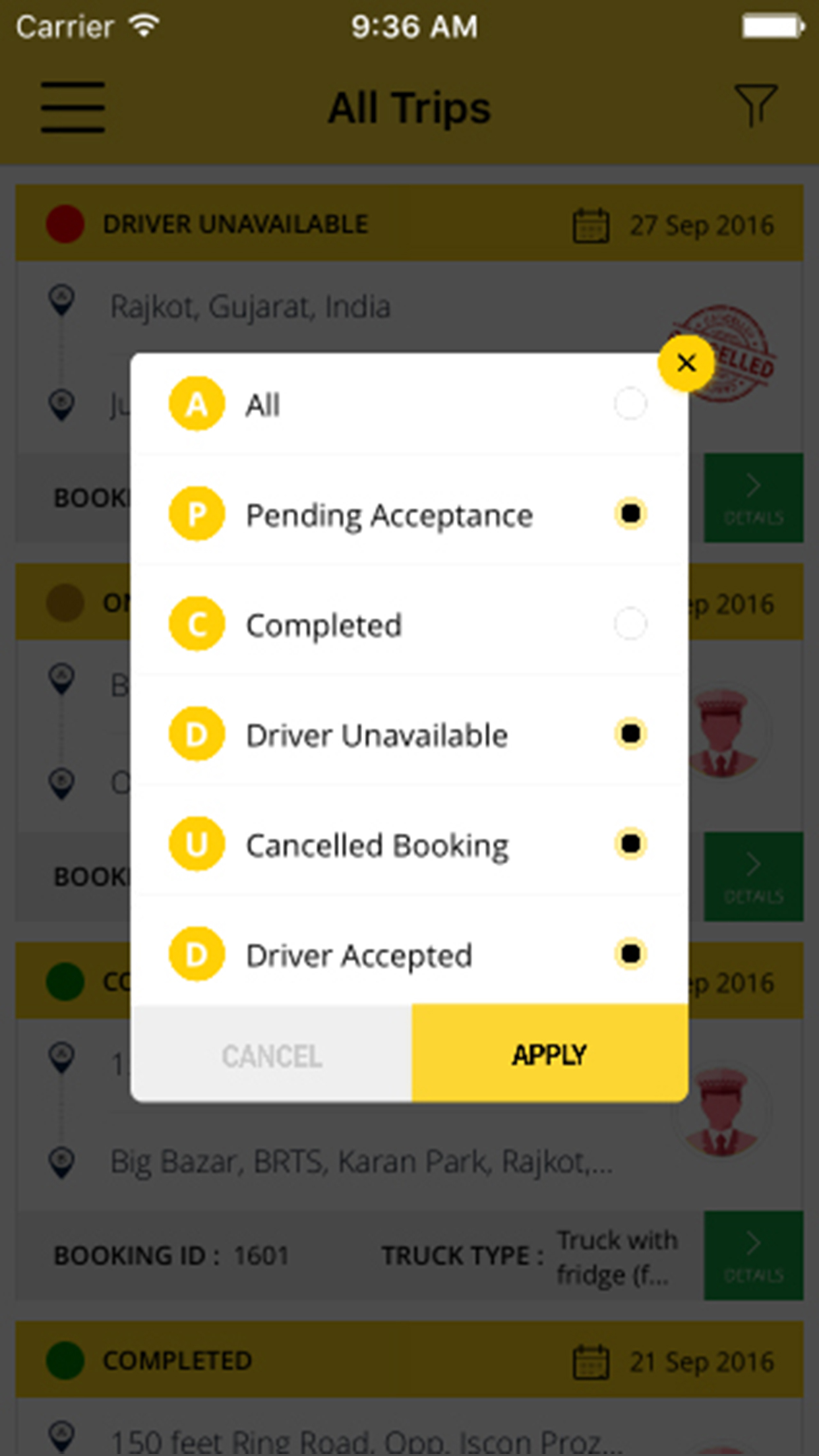The image is a screenshot from an iPhone displaying an app related to car and truck ride bookings. The app features a predominantly yellow color scheme, with a yellow banner at the top containing a hamburger menu and the text "All Trips." Below the banner, the first entry on the screen is marked with a red circle and the text "Driver Unavailable," dated September 27, 2016.

In the foreground, a pop-up window obscures much of the background. This pop-up is brightly lit compared to the dimmed background and features a yellow circle with an "X" in the upper right-hand corner for closing it. The pop-up contains a list of selectable options, presented in order from top to bottom as follows: "All," "Pending Acceptance," "Completed," "Driver," "Cancel Booking," and "Driver Accepted." The options "Pending Acceptance," "Driver Unavailable," "Cancel Booking," and "Driver Accepted" are ticked, indicating they are selected. At the bottom of the pop-up, there is a yellow "Apply" button with black text.